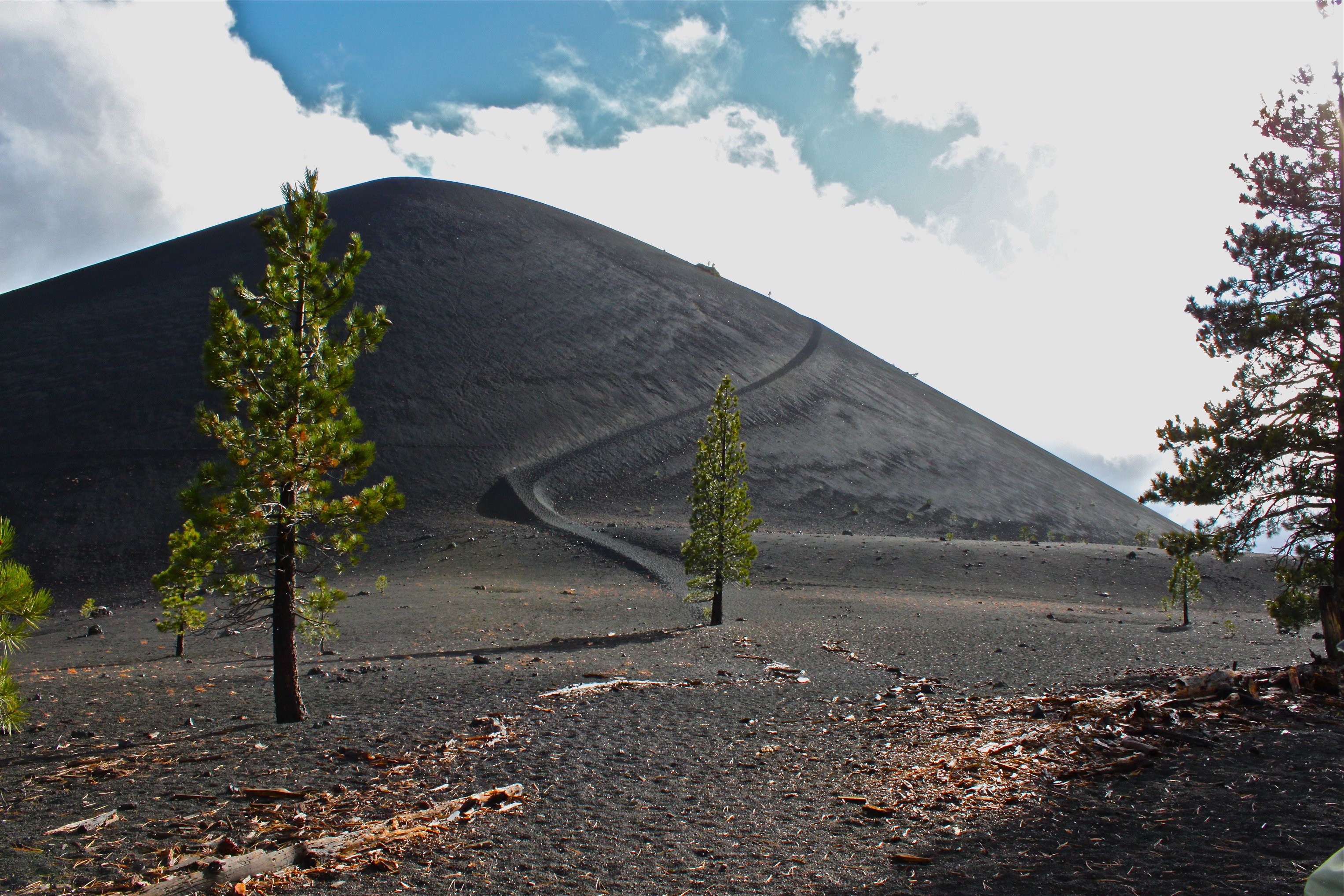This photograph captures an outdoor scene marked by a stark, desolate beauty. Dominating the background is a large, black hill, its color potentially the result of volcanic activity or some kind of burning, giving the landscape an eerie, scorched appearance. Above, the sky is a brilliant blue, scattered with an array of fluffy clouds, suggesting a bright afternoon with the sun high and hidden behind the clouds. The foreground features five tall, slender coniferous trees, reminiscent of Christmas pines, which appear newly planted in an otherwise sparse and barren terrain. The ground is dark, contrasting sharply with light tan wood shavings scattered beneath the closest trees, possibly remnants of the past destruction. A narrow, winding road or path can be seen weaving its way up the hill, leading towards indiscernible structures or objects that add an element of mystery to the scene. This picture exudes a haunting, yet strangely captivating, blend of natural and post-apocalyptic beauty.